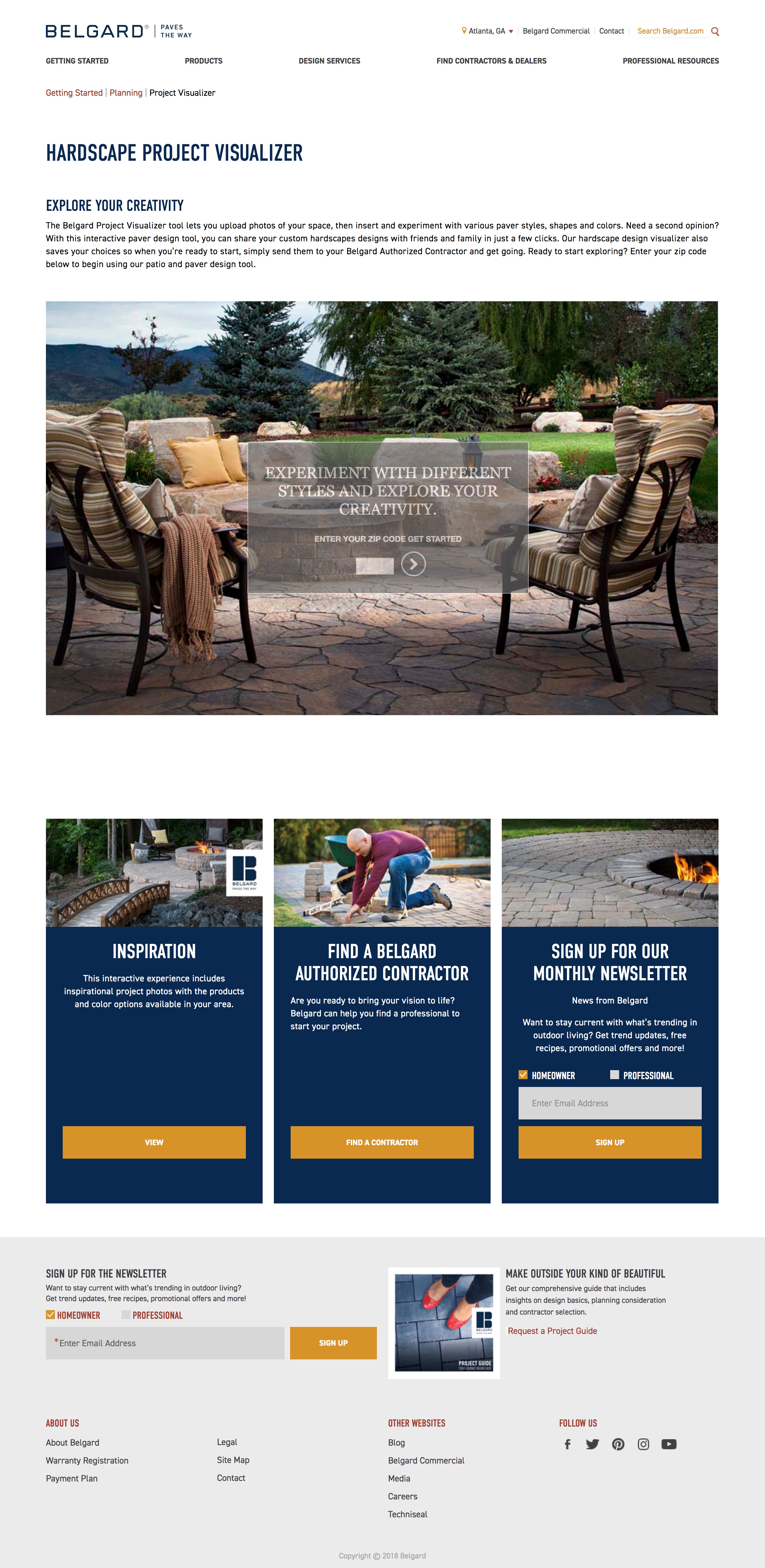This image displays a screenshot of a website with a clean, white background. At the top, the header prominently features the logo "Belgard" in bold text, followed by their tagline "Paves the Way." To the right, navigation links read: "Atlanta, Georgia," "Belgard Commercial," "Contact," and "Search belgard.com."

The main navigation menu includes links to several sections: "Getting Started," "Products," "Design Services," "Contractors and Dealers," and "Professional Resources." Below, a sub-navigation again emphasizes "Getting Started," featuring links titled "Planning" and "Project Visualizer."

The main content of the page introduces the "Hardscape Project Visualizer" in large, capitalized text. Below this title, slightly smaller but still prominent text reads "Explore Your Creativity," followed by a descriptive paragraph. The page features a scenic outdoor image showcasing a serene atmosphere with sky, mountains, trees, a lawn, and a stone patio furnished with outdoor furniture. Overlaid text on this image encourages users to "Experiment with different styles and explore your creativity." A call-to-action invites users to enter their zip code to get started, indicated by a circular icon with a right-facing arrow.

Further down the page, three additional visuals highlight three actions: "Inspiration," "Find a Belgard Authorized Contractor," and "Sign Up for Our Monthly Newsletter."